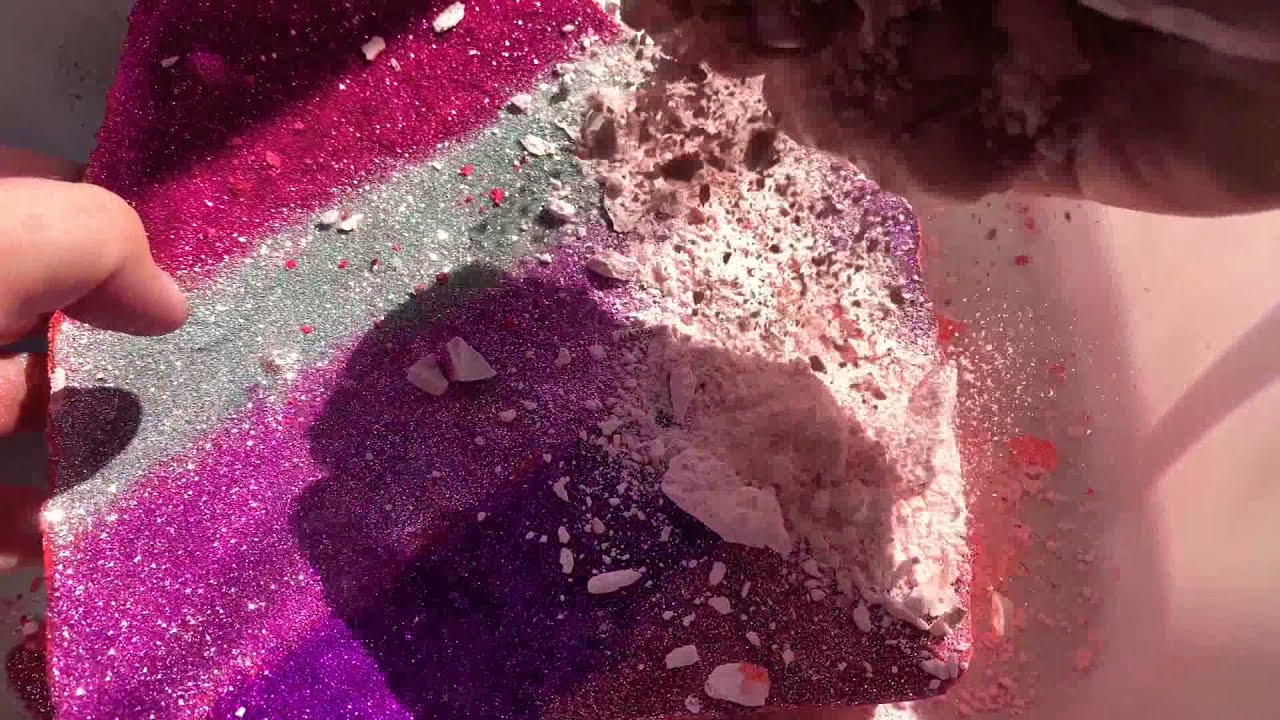In this close-up image, we see a person, likely a woman, engaged in an intricate art project. The setting is ambiguous, potentially indoors or outdoors, but it’s clear that creativity is at work here. On the left side of the image, her hand is visible, delicately holding a broken stone, with a few of her fingers slightly in view. The main focus is a central broken stone, its fragments scattered around, revealing a complex array of colors: dark pink, fuchsia, gray, purplish tones, white, and tan. The background blushes with a pale pink hue. Smaller rock pieces, tinted red, are sprinkled near the right side of the image. This scene could also involve elements of glitter, mistakenly perceived as minerals, contributing burgundy, silver, gray, pink, and very purple hues, giving the appearance of glittery artwork. The overall array of colors and textures creates a captivating and vibrant visual medley.